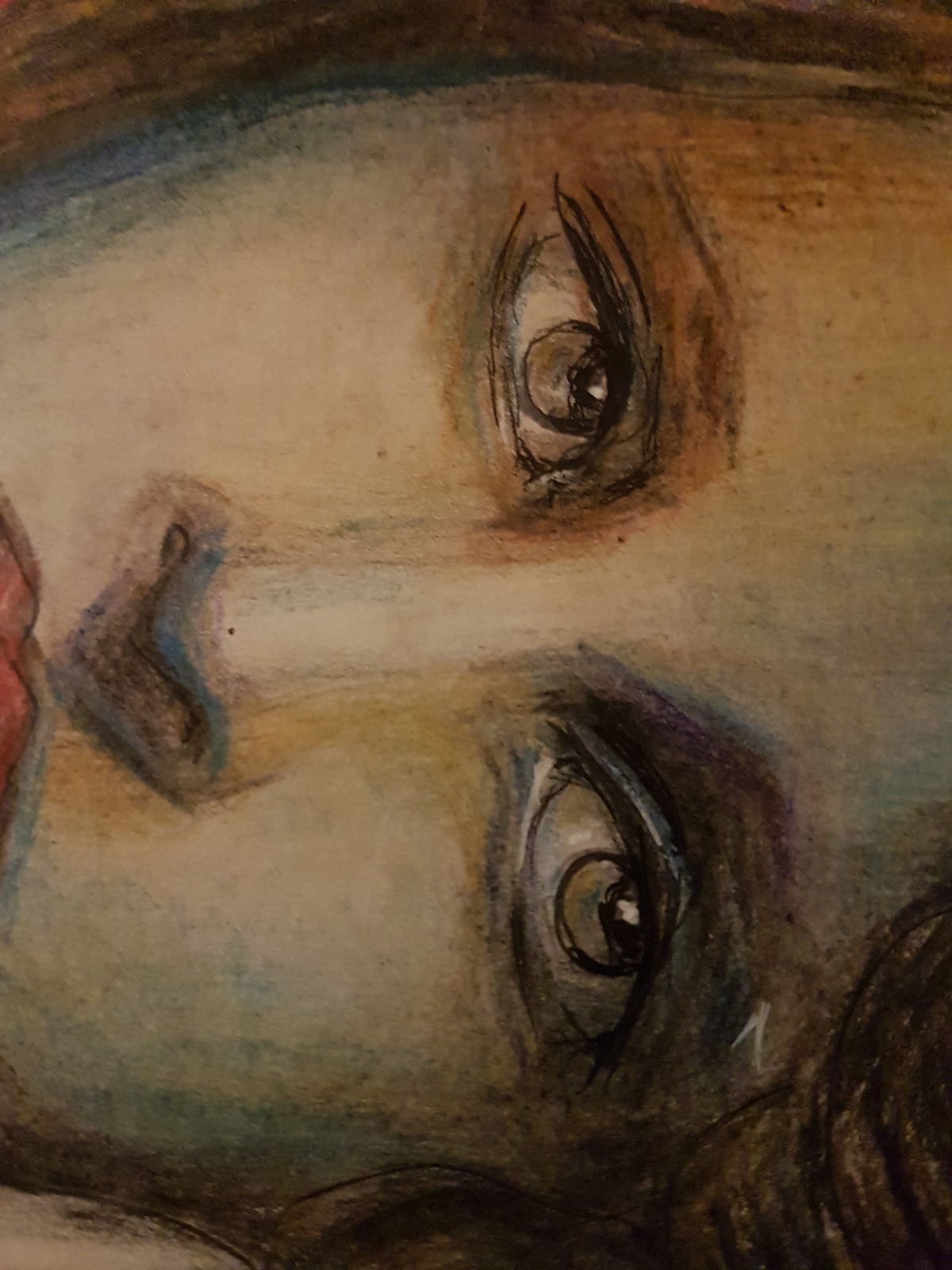This image captures a detailed drawing of a woman's face in a rectangular frame oriented with the longer side from top to bottom. The face appears sideways, suggesting the woman is either lying down or the drawing was rotated. The visible features include primarily the eyes, nose, and the top portion of her lips. 

The woman, portrayed as Caucasian with a light cream complexion, seems to have a somber expression with deep-set, light gray eyes. Her pupils are black, and she gazes slightly upwards and to the right. The eyebrows are not well-defined, and there are shadows and hints of browns and grays around her eye sockets, hinting at a melancholy or contemplative mood. The nose is long and thin, casting a shadow at the bottom, and ends in a loose W shape. 

Only the top of her lips is visible, highlighted in a bright red with a perfect Cupid's bow. A small amount of curly brown hair frames the bottom corner of her face. The entire image is predominantly painted in brown tones and is devoid of other significant details, focusing entirely on the expressive and shadowed features of the woman's face.